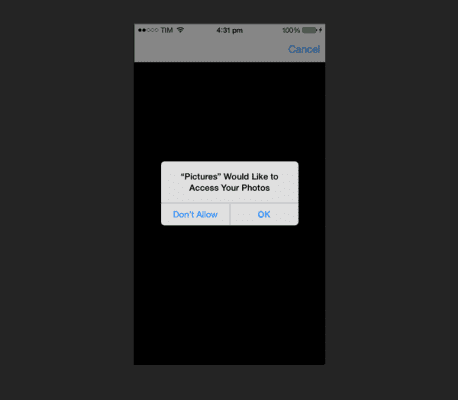This image features an iPhone displaying a screenshot within the Photos app. The central focus is a white dialog box that prompts the user for permission to access their photo library. The message reads: "Pictures" would like to access your photos. Below this message, two options are provided: "Don't Allow" on the bottom left and "OK" on the bottom right, both in blue text. Selecting "Don't Allow" will deny access, while clicking "OK" will grant it.

The screenshot is framed by a dark gray border. The primary background of the iPhone's display is black, providing a stark contrast to the white dialog box. 

At the top of the iPhone's screen, several status indicators are visible. On the left side, the phone's signal strength is shown along with the carrier name, "TIM." Centered at the top, the current time is displayed as 4:31 PM. On the right side, the battery level shows 100%, accompanied by a lightning bolt icon, indicating that the phone is currently charging. Additionally, just below the battery indicator, there is a blue "Cancel" option, which would abort the current action and return the user to the previous screen.

The overall layout of the screenshot highlights the dialog box effectively, emphasizing the user's choice to manage photo access permissions.